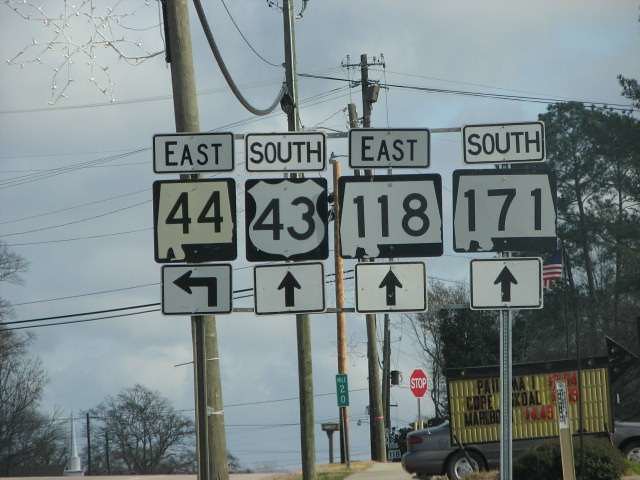This color photograph captures a cluster of four street signs prominently displayed on a silver L-shaped post, set against a backdrop of a general outdoor landscape with a gray, overcast sky. Starting from the left, the first sign reads “East” on a small rectangle above a square sign displaying the number “44” with a left-pointing arrow below it. The next sign says “South 43” with a straight arrow underneath, followed by another sign stating “East 118” with a straight arrow. The final sign on the right reads “South 171” with a straight arrow. Beneath these main directional signs, there is a smaller movable road sign with illegible black lettering on a yellow background. The scene also features telephone poles stretching into the distance, a stop sign, a parked car, and a church steeple. Festive snowflake Christmas lights adorn the pole in the foreground, adding a seasonal touch to the otherwise dreary day.